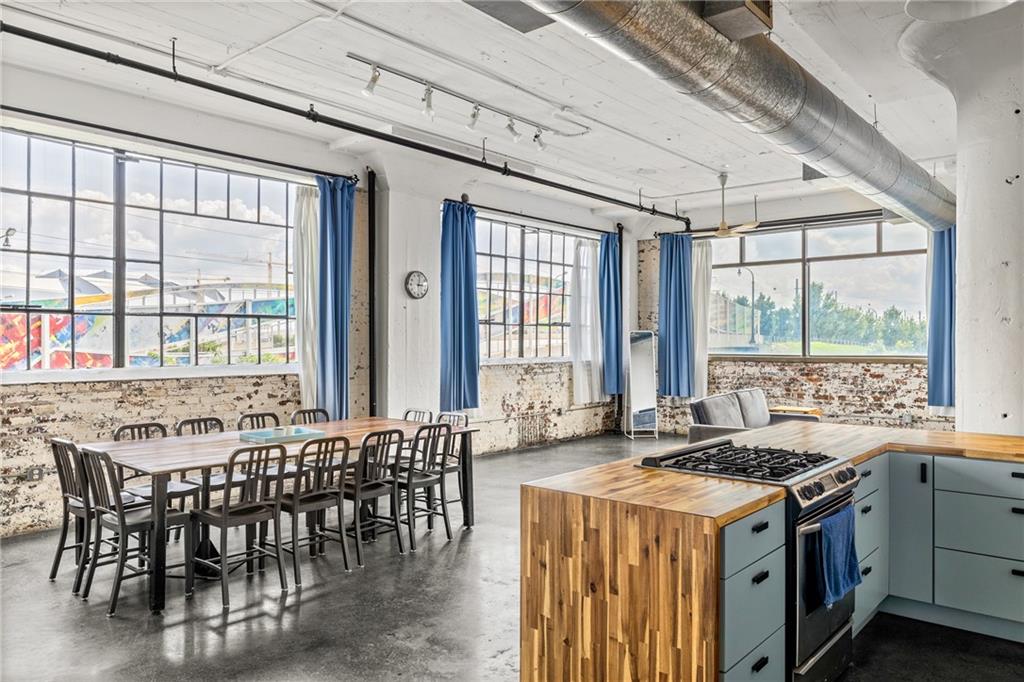This is a detailed photograph of a spacious kitchen with a weathered charm. The floor is a dark green slate, adding depth and richness to the room. Dominating the center, there is a large wooden and metal-framed table surrounded by 12 gray metal chairs, suggesting it’s designed for large gatherings. The table and chairs have a robust, industrial feel.

To the right, there's a substantial brown wooden countertop that hosts a central cooktop with elevated burners, suggesting a gas range. Beneath this countertop are many white cabinets with black handles, alongside an oven from which a blue towel hangs. Above the counter, the walls are made of weathered white-painted brick, with patches of natural brown brick showing through, adding a rustic touch. 

The kitchen has ample natural light streaming through its large, square-paneled windows, adorned with blue and white curtains pushed open, on both the front and right walls. Additional features include a tall mirror in the corner and a round clock on the wall, both enhancing the room's character.

The ceiling is white and houses an exposed HVAC pipe for ventilation, along with unlit light fixtures. In the background, a gray loveseat is partially visible, suggesting an open-plan design extending into a living area.